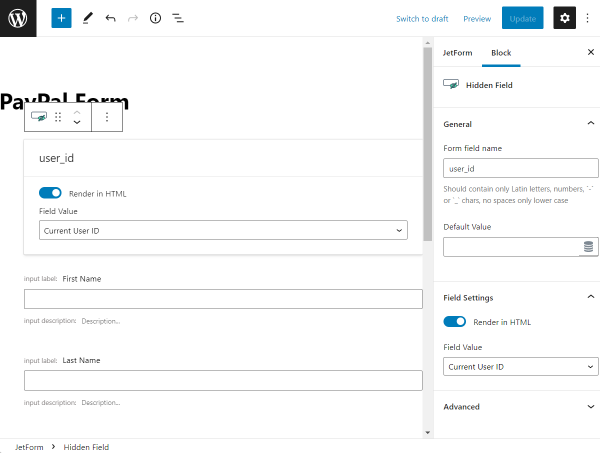The screenshot depicts a web form interface with overlapping elements, causing partial obstruction of the header section by an information box. The visible portion of the header likely reads "PayPal Form." Below this is a section labeled "User_ID" along with the text "Reminder to render in HTML," accompanied by a toggle button. The field labeled "Current User ID" displays a value, while the "First Name" and "Last Name" input boxes are empty. 

On the right side, the interface displays another form context titled "Chat Form and Block". This section includes a field labeled "General Form Field Name" with the value "User_ID", followed by default settings and field values, mirroring those on the left side. Overall, the interface appears to be a form editor or builder with customizable fields and settings.